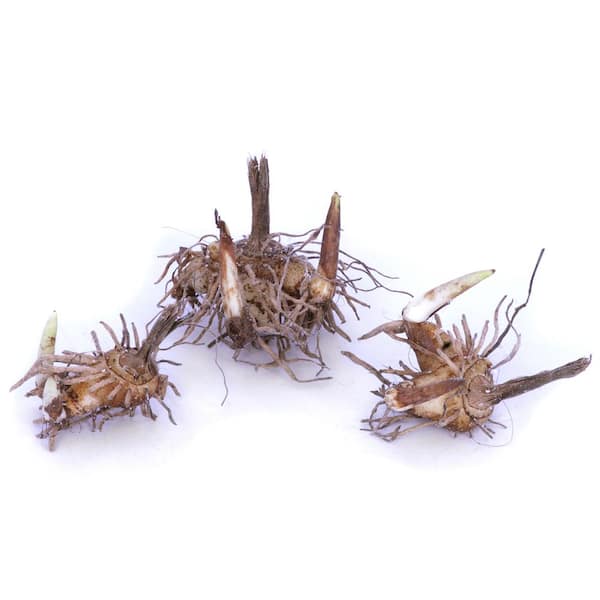This photograph showcases three distinct organic arrangements that resemble seed pods or abstract representations of small creatures, situated against a stark white background. Each arrangement comprises a cluster of thin, brownish tendrils radiating in a ring pattern from a central, larger stem, creating an intricate display that hints at dried roots or branches. The clusters are positioned symmetrically with one in the center and two on either side. Each formation features interwoven wiry branches and sticks, blending shades of brown and light brown, and casting delicate gray shadows below. The overall composition of each object evokes the likeness of small, abstract creatures such as bugs or birds, formed from the tangled and crisscrossing natural elements.